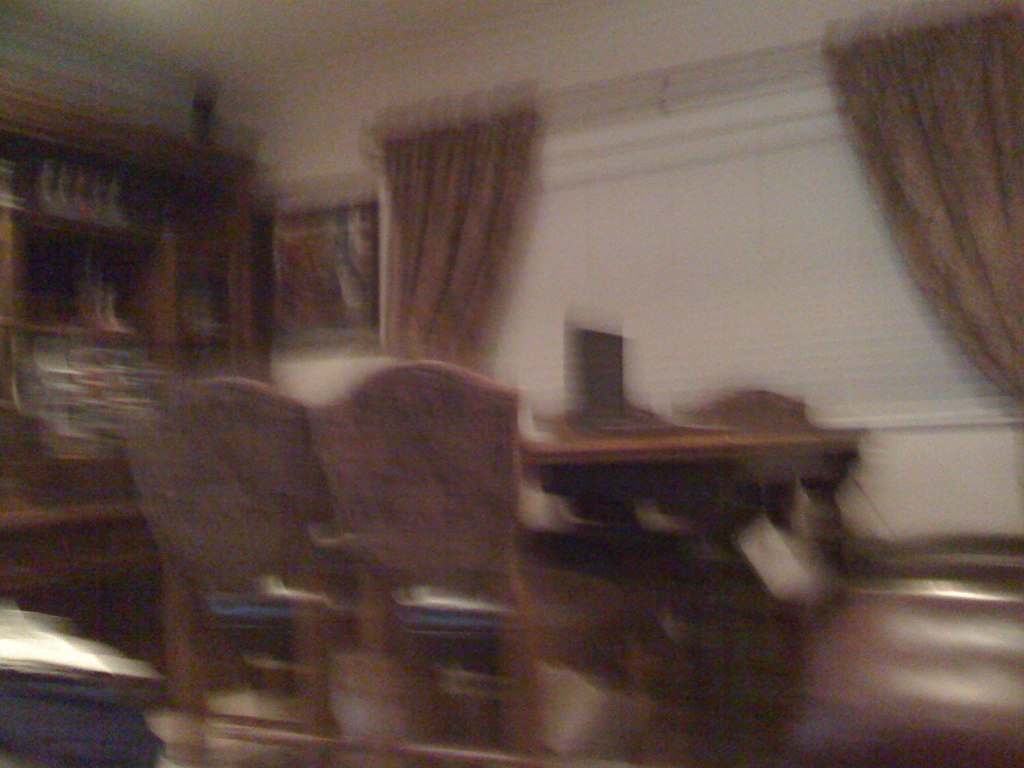The image portrays a dining room, captured from a first-person perspective. The photograph is of poor quality, being both blurry and grainy, suggesting motion during the capture and a lower quality camera. The main focus is a brown wooden table with two wooden chairs in front, each upholstered with blue cushions. Behind the table, there is a large window with white mini blinds, partially obscured by thick brown curtains pulled off to the side. To the left of the window, a dark-framed piece of wall art with hints of blue and white can be seen. Adjacent to the art is a brown curio cabinet, vaguely revealing white stick figure decorations inside. Nearby, a dark blue and white object is vaguely visible, and to the right of the table, there is a seating area, possibly upholstered in maroon-colored leather. On top of the table, a rectangular object resembling a laptop or a book is present. The overall composition suggests a dining area shared with other pieces of furniture, highlighted by the characteristic poor quality of the image.